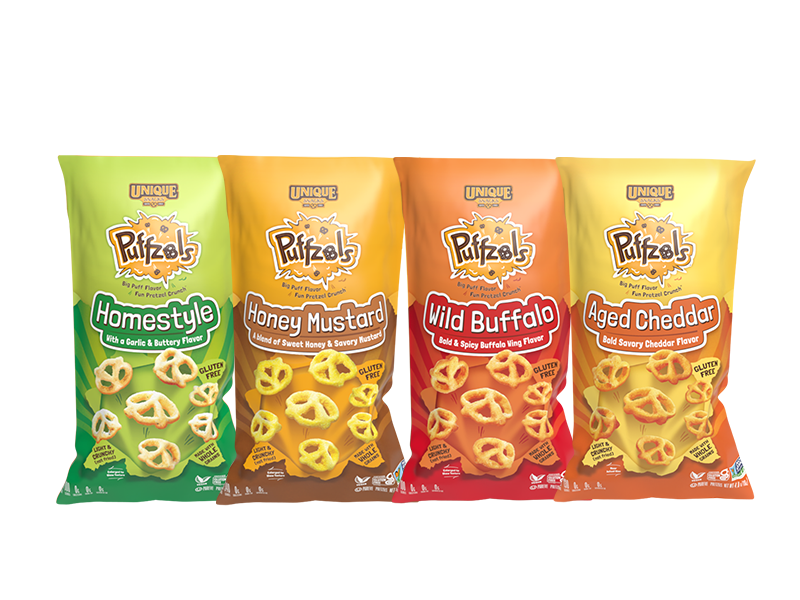The image displays four vividly colored bags of snacks called "Puffzles," each corresponding to a unique flavor and organized horizontally against a white background. From left to right, the first bag is green and dark green, labeled "Home Style" with a garlic and buttery flavor. Next is the beige and brown bag of "Honey Mustard," offering a blend of sweet honey and savory mustard. The third bag, in shades of orange, dark orange, and red, features the "Wild Buffalo" flavor, described as bold and spicy. The final bag is yellow and orange, marked as "Aged Cheddar," which promises a bold and savory cheddar taste. Each bag prominently displays the brand name "Unique" at the top, along with images of puffed, pretzel-like snacks beneath the flavor description.